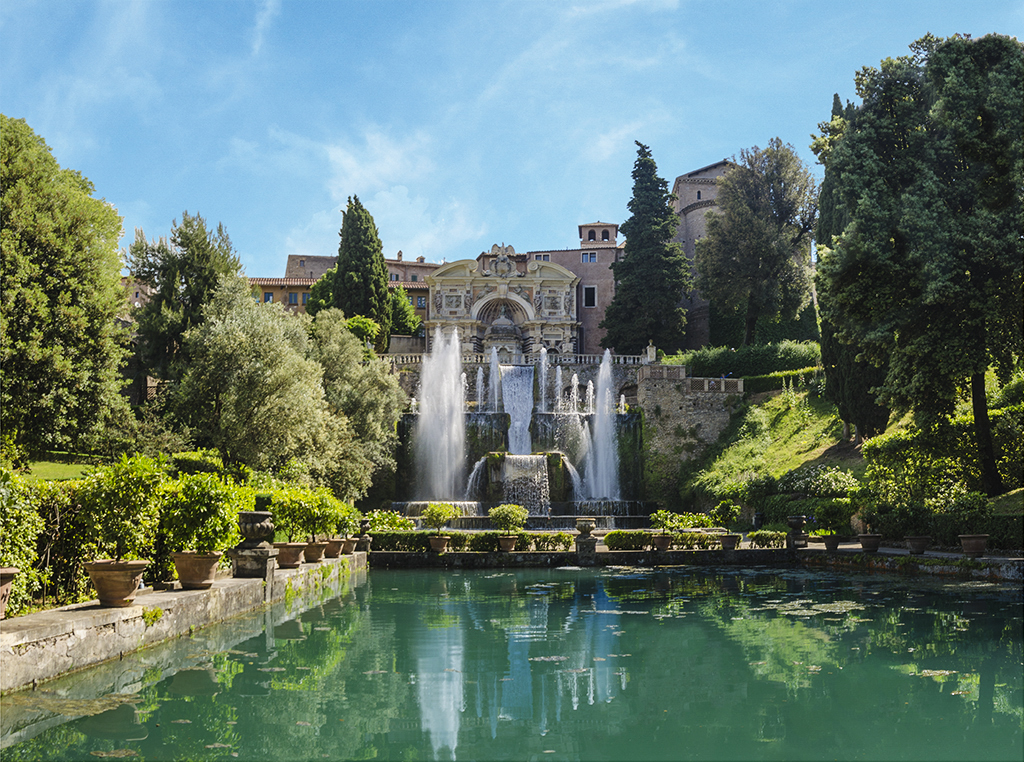In this stunning outdoor image, a magnificent mansion—resembling a castle—commands attention from its elevated position atop a hill. The mansion features large tan columns and a blend of brownish and tannish hues in its multi-level, sprawling structure. Surrounding the mansion are meticulously manicured green hedges and trees that enhance its grandeur. In the foreground, a vibrant green-blue pool, likely painted for effect, reflects the surrounding flora and various shadows. Numerous potted miniature orange citrus trees encircle the pool, adding to the lush scenery. Beyond the pool, two main fountains and several smaller ones send streams of white water skyward, creating an elegant water display. The primary building boasts light pink walls and black windows, with a fancier central structure in light yellow, set against a backdrop of clear blue skies with minimal clouds.